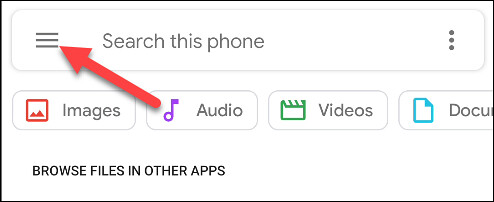The image captures a screenshot of a phone screen, specifically from an information or instructions page. At the top of the screen, there is a search bar prominently displayed. On the left side of this search bar, there is a "hamburger" menu icon (three horizontal lines), with a large red arrow pointing towards the bottom right of the icon. Inside the search bar, the text "Search this phone" is visible. On the right-hand side of the search bar, there are three vertical dots, indicating a menu for additional options or settings.

Below the search bar, there are four horizontally aligned buttons. The first button, labelled "Images," includes a small red icon depicting an image. To its right, the "Audio" button features a purple music note icon. The "Videos" button follows, adorned with a green clapperboard icon. The last button, partially cut off in the image, is labelled "Documents" and includes a blue document icon.

Under these buttons, there is some text reading "Browse files and other apps." On the far right-hand side of the screen, there is an icon that appears to be related to help, edit, or some form of troubleshooting, though its exact purpose is unclear from the screenshot.